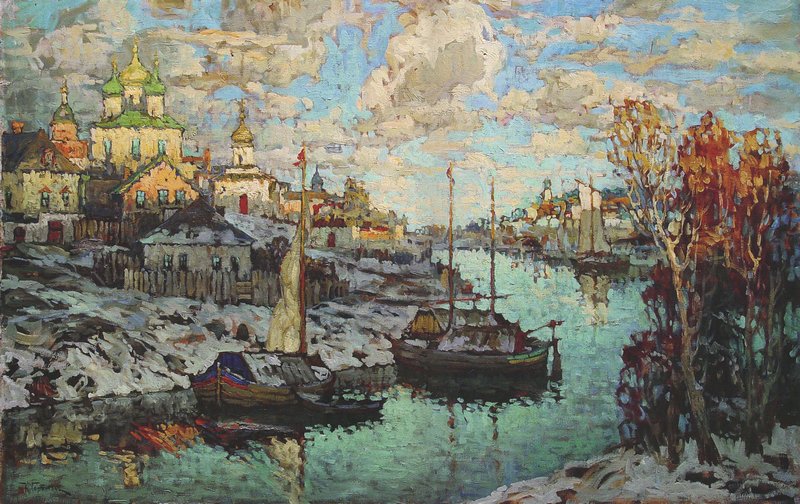This painting captures a tranquil winter scene in a historical seaport town. At the center of the image is a small river, depicted with a mix of green and blue hues, reflecting the surrounding environment. Numerous sailboats are docked on the river, adding to the serene waterfront atmosphere. The riverbanks are dotted with trees, some bare while others display autumn leaves in vibrant red and orange. Snow covers the ground, amidst scattered dead leaves, indicating a transitionary period between fall and winter.

The background of the painting is dominated by an array of buildings, including one with distinctive triple spires, reminiscent of Russian or Greek Orthodox architecture. Another notable building has a green roof, contributing to the multicolored landscape that also features diverse shades of blue, gray, white, green, orange, red, and tan. The sky, occupying the upper portion of the painting, is mostly cloudy with patches of blue, suggesting a late afternoon with the sunlight fading and casting the foreground in shadow while illuminating the distant buildings.

In the bottom right corner, there appears to be a signature from the artist, subtly confirming the painting's authenticity. The artist has skillfully captured the reflective qualities of the water and the intricate details of the town, making this piece a potential highlight in any art show.